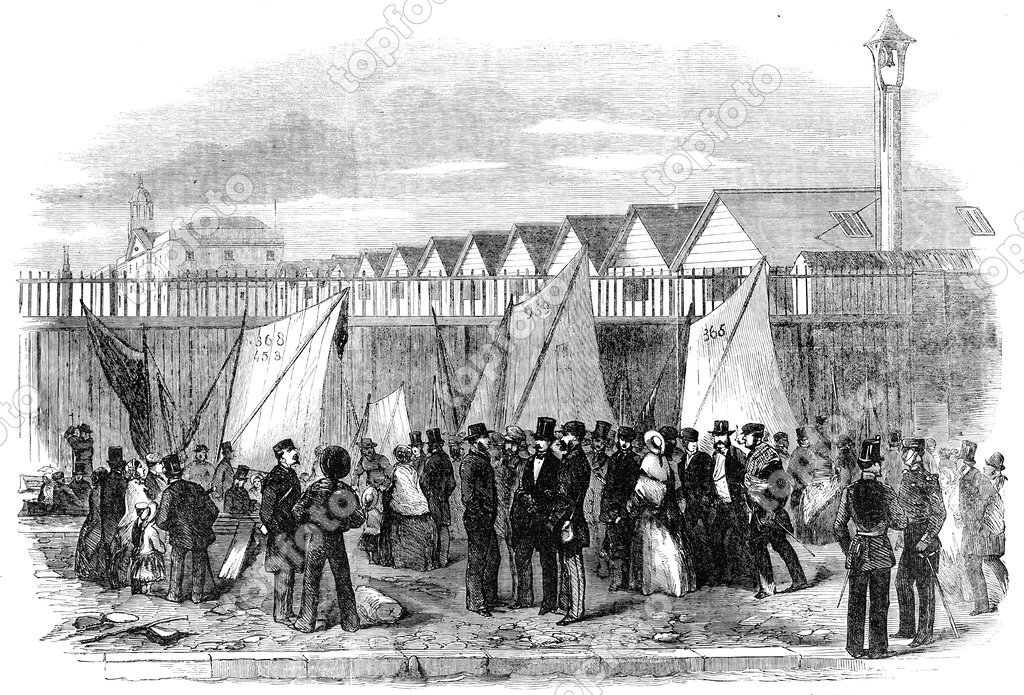This black-and-white pencil illustration, marked repeatedly with the "TOP FOTO" watermark, showcases a Victorian-era street scene, likely from the 1800s. In the foreground, a gathering of people dressed in period-appropriate clothing is depicted. The men are attired in black top hats and suits, with some appearing to be military officers holding swords at their waists, while the women wear sun hats and long dresses. To the right, a tall street lamp stands lighter in color compared to the other elements. Additionally, several policemen with hats can be seen on the corner. Behind the assembly, a tall wooden wall is visible, with raised white fabrics supported by poles, displaying faint and unclear numbers such as 368403, 969, or 366—resembling tents. In the background, rows of wooden bungalows with triangular roofs are depicted, alongside a large mansion with a central tower. The scene provides a detailed glimpse into a bustling Victorian street life.